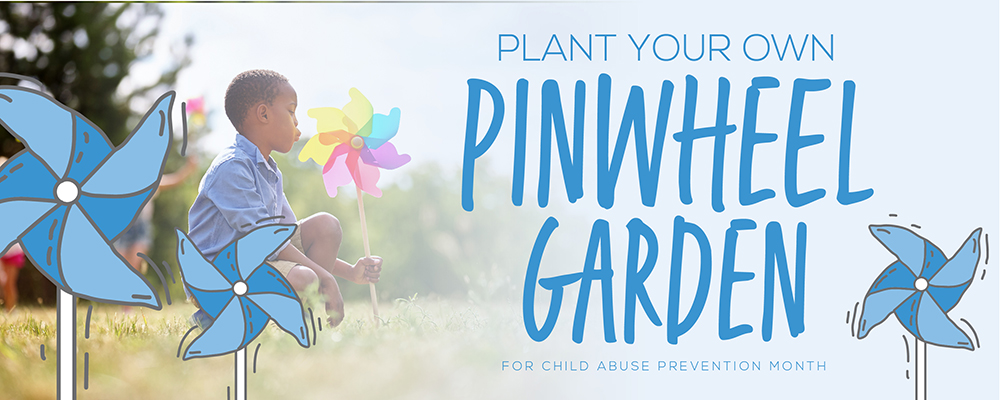This ad is a combined illustration and photographic design, promoting Child Abuse Prevention Month with the call to "Plant Your Own Pinwheel Garden." The primary text is in clean, modern blue font with the words "Pinwheel Garden" styled in a handwritten marker font. The ad features three cartoon pinwheels in shades of blue, drawn to convey motion with lines suggesting they are spinning in the wind. The background transitions from a vibrant scene to a light blue gradient that hosts the text on the right-hand side.

Central to the image is an African-American boy with dark skin and a blue shirt, squatting in a grassy field with some trees nearby. He is blowing on a colorful rainbow pinwheel with petals in yellow, blue, pink, red, and purple, creating the illusion of motion. The vibrant boy's image is juxtaposed with the serene background, where faint figures and trees can be spotted, partially obscured by the illustrative pinwheels. The thematic blue tone is consistent throughout the piece, enhancing the visual connection between the various elements of the ad.